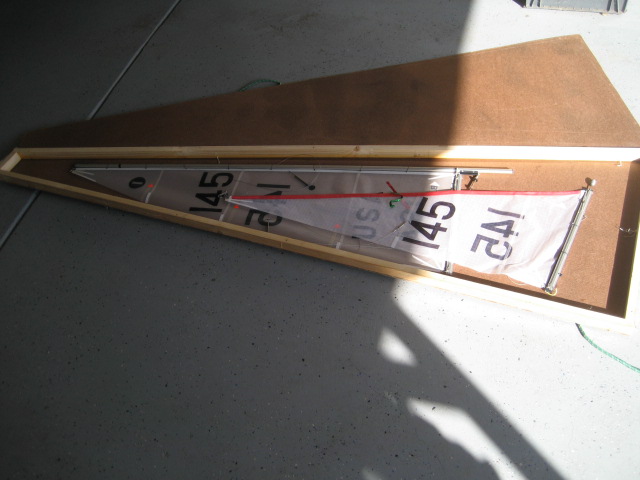The image features a large measuring device, likely used for sports fields, centrally positioned on a plain, white-tiled surface. The device has a triangular shape and is constructed from two connected pieces of particle board-like material. In the center of one section, numbers "145" are printed on small plastic plates. The photo exhibits strong contrast in lighting, with the right side bathed in bright sunlight and shadows covering about two-thirds of the left side. Additionally, a green mark is visible on the floor.